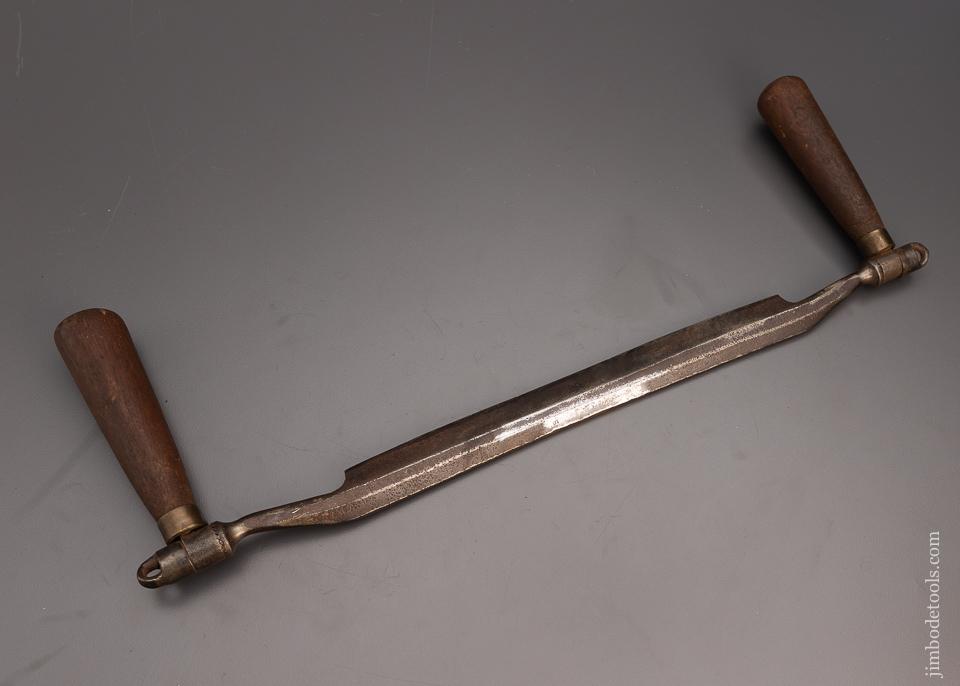This photograph, set against a brownish-gray background, depicts an antique agricultural tool, likely a thatcher or similar scythe-like instrument designed for cutting plants. The image features a long, slightly tarnished metal blade running diagonally from the lower left to the upper right corner, with some patches of shining silver in the center and rust on the edges. The blade is connected to two dark brown, well-worn wooden handles positioned vertically at each end, each adorned with a gold or copper cap where they attach to the blade. The handles show signs of age and use, hinting at the tool's history and functionality. In the lower right-hand corner of the image, white vertical text reads "JimBodeTools.com," suggesting a source for further information about the tool.